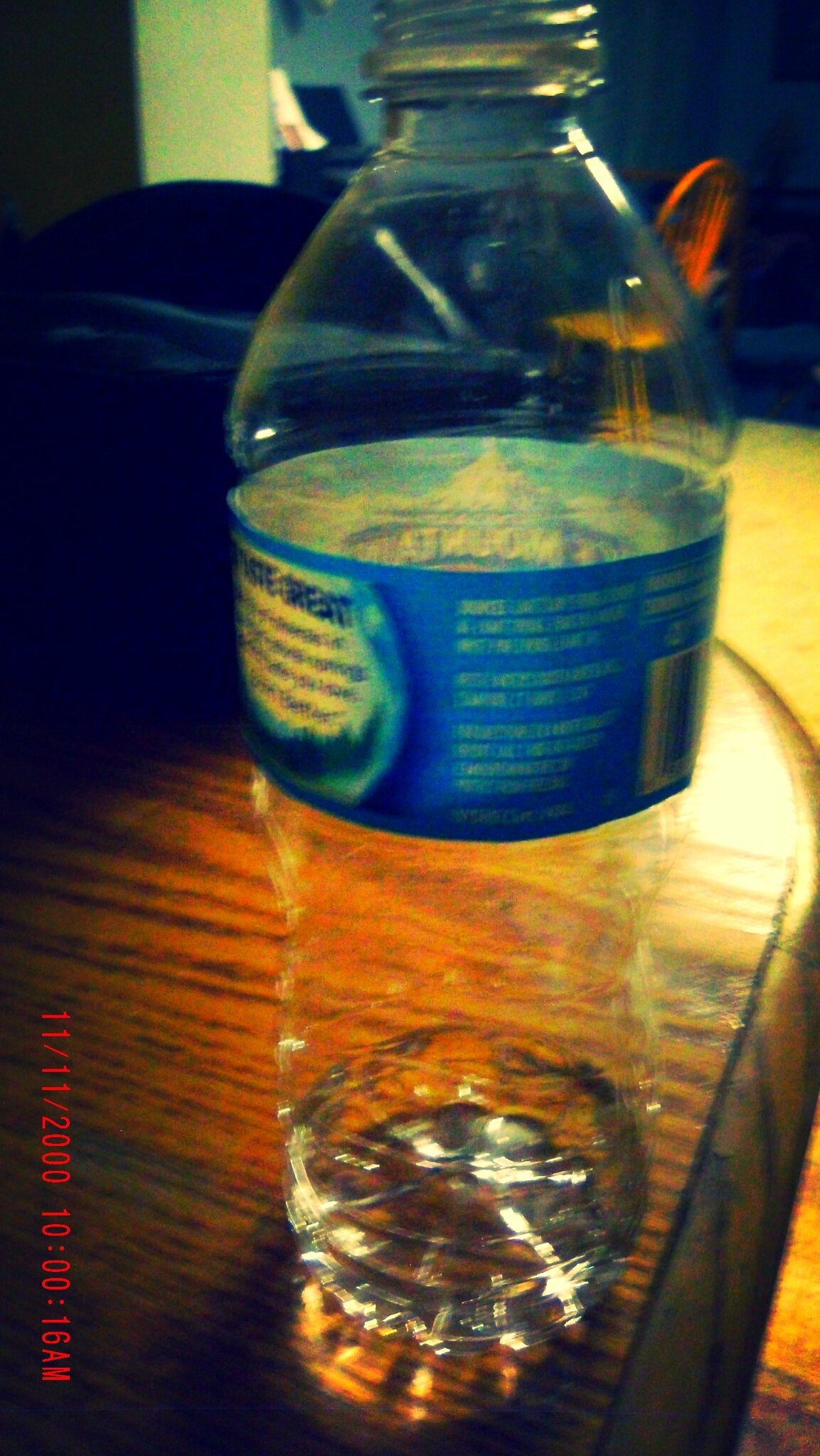This vertically oriented rectangular image, which lacks a border and is slightly blurry, features a central focus on an almost empty plastic water bottle with a blue and white label. The bottle is positioned towards the middle of a medium brown wooden table with dark wood grains. The cap is missing, revealing the rim where it would screw on. The label on the bottle indicates a brand name containing the word "mountain." In the lower left-hand corner of the image, there is a timestamp vertically printed: "11/11/2010 16 a.m." The background reveals a red chair with a wooden seat and possibly a second chair or a couch, which is either black or navy blue. Among the array of colors in the scene are shades of red, blue, light blue, gray, and orange. Additionally, a black bag can be slightly seen on the table. The photo is taken indoors, presumably in a household, with various objects subtly included but indistinct due to the blurry focus on the water bottle.